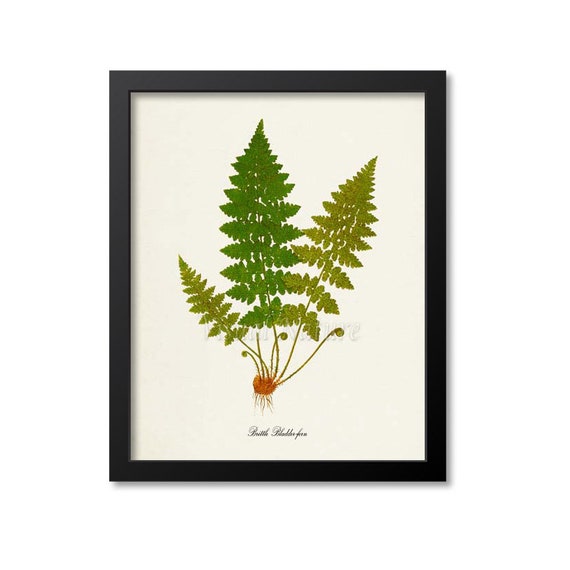This image, set against an all-white background, features a photograph of a framed botanical illustration. The black frame encloses an elegant print depicting a fern plant in meticulous detail. The central focus is on three fern fronds: the largest one in the center, a medium-sized one extending to the top right, and the smallest reaching towards the top left. These fronds exhibit a spectrum of green shades, from dark green to light yellow-green, capturing the delicate, lacy appearance reminiscent of Queen Anne’s lace.

At the base of the ferns is a reddish bulb, adorned with roots that dangle from it, some entwined with brown dirt. Several stems emanate from this bulb, with some curling upwards, showing both mature fronds and budding stems. The lower part of the picture contains blurrily-rendered cursive text, with a watermark reading "Visual Nature." This thorough depiction captures the fern's entire structure, from the intricate leaves to the detailed root system, all set within a sleek, basic black frame on a pristine white wall.